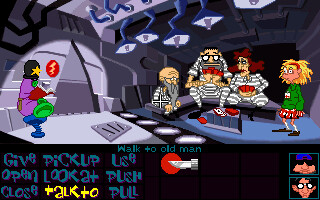The image is a detailed screenshot from a video game resembling a comic strip, set in a futuristic gray interior. The scene depicts a decision-making interface at the bottom, featuring options like "give," "pick up," "use," "open," "look at," "push," "close," "talk to," and "pull," with "talk to" highlighted in yellow on a black background. Towards the top, "walk to old man" is displayed in blue text. 

The setting appears to be a jail or holding area, populated with various characters. On one side, an old bald man with a long gray beard sits on a couch next to a man with black hair and glasses, both dressed in black and gray striped clothing, playing cards with a woman who has red hair and is also holding cards. Nearby, a girl with striking blonde-red hair, wearing a green shirt and a red-and-black checkered skirt, stands out with her white socks and black shoes. 

To the left, a figure wrapped in gauze sits on a stool, while on the right, there's another mysterious character wearing a kimono-like outfit, colored purple and green with a gold star, sitting on a blue chair. The visual style, with its angled and uniquely shaped lighting, enhances the comic strip aesthetic, emphasizing the cartoon-like appearance of the characters and environment.